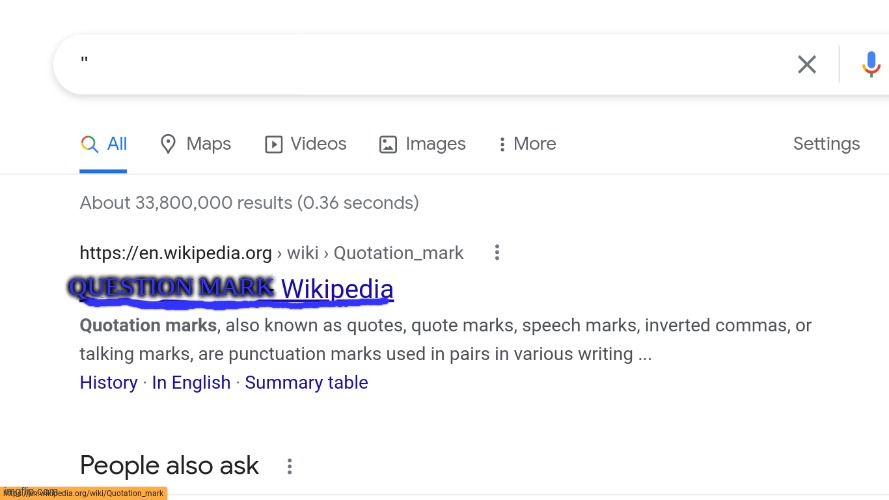An image depicting a Google search results page, with a search box at the top containing only a pair of parentheses. The distinct colored microphone icon is visible on the right side of the search box, indicating the use of Google's search engine. The search yielded 33,800,000 results in 0.36 seconds. The first result displayed is the Wikipedia entry for "quotation mark," with the hyperlink to the Wikipedia page highlighted and a blue question mark overlaid on the link text. The bottom left corner of the image shows the "People also ask" section in black text. The background of the webpage is entirely white, providing a stark contrast to the elements on the screen.